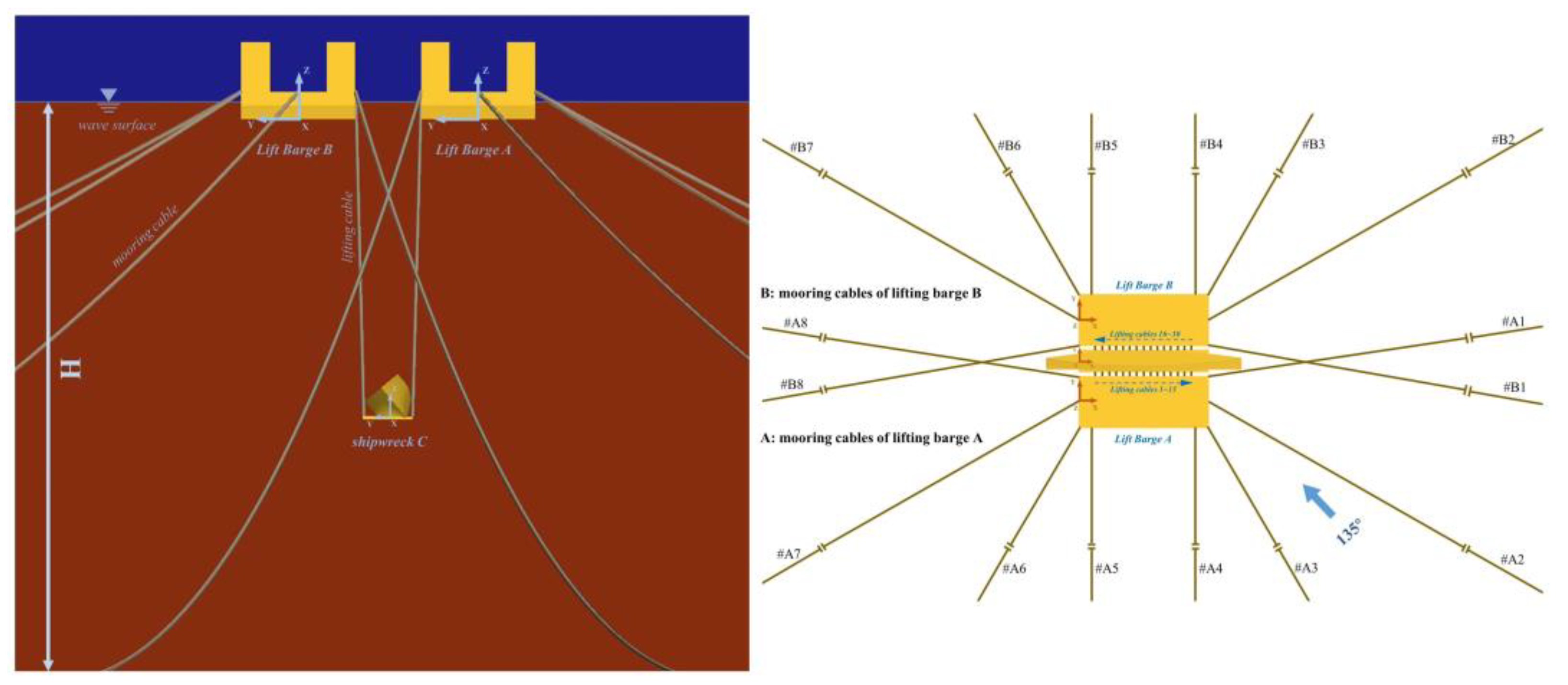This image comprises a detailed two-part diagram illustrating the configuration of mooring cables for lifting barges A and B during a shipwreck salvage operation. The left side of the image features a pair of yellow, U-shaped structures labeled as Lifting Barge A and Lifting Barge B, which are connected to a sunken object via numerous cables. These cables fan out from the top of the diagram towards the barges in various directions, resembling bridge cables, and are drawn over a background that transitions from dark blue at the top to red at the bottom. The right side of the image presents a more intricate view focused on a single barge, detailing the angles and labels of each of the cables extending from it. The entire setup appears to serve as an instructional guide, likely akin to a manual or computer training program, with the primary colors being yellow, red, and greenish-blue. The text accompanying the cables identifies them as "mooring cables of lifting barge A" and "mooring cables of lifting barge B," reinforcing the instructional nature of the diagram.